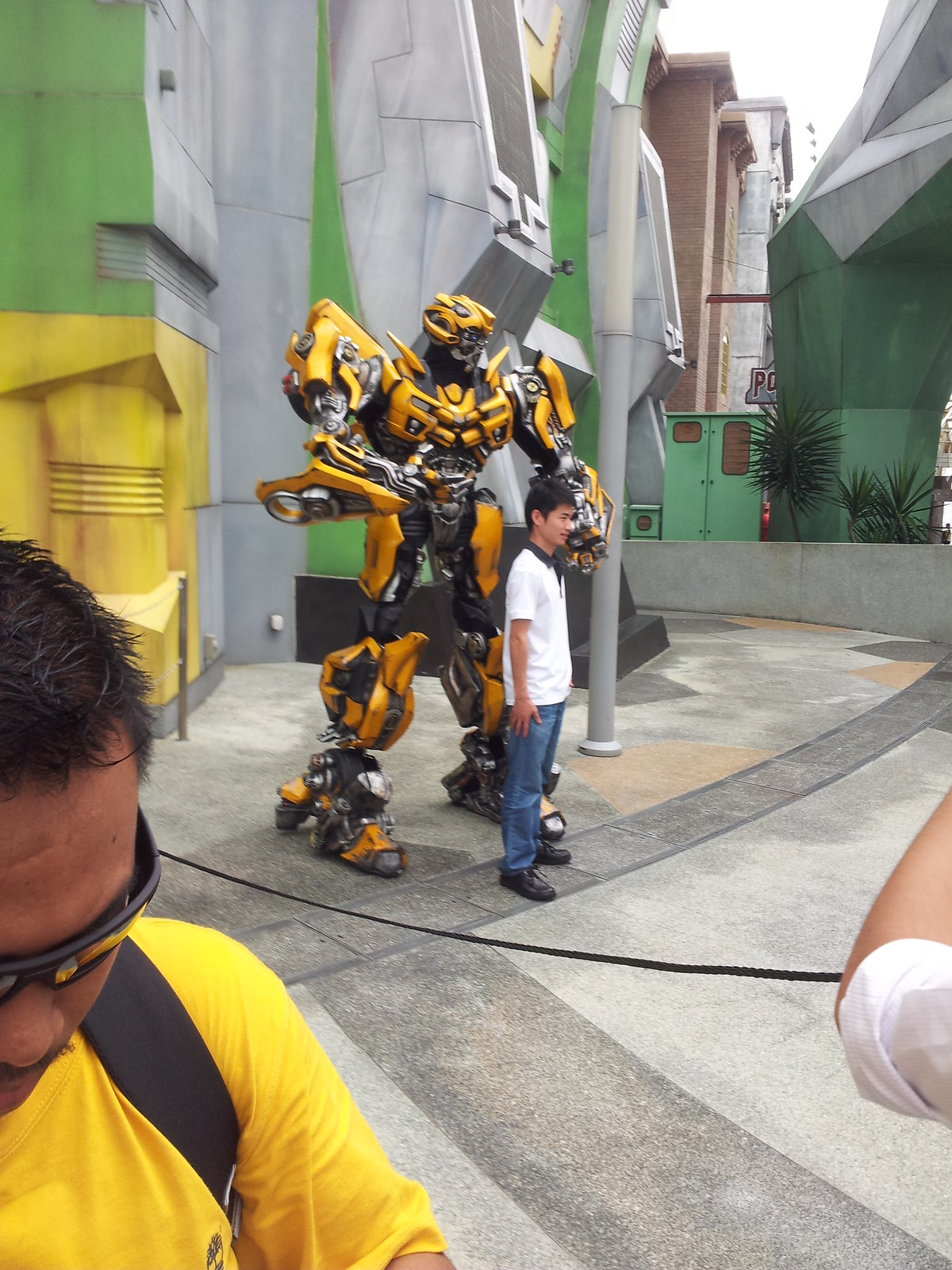The photograph features a young Asian man, likely in his late teens or early 20s, with short black hair, wearing a white t-shirt, jeans, and black sneakers. He is posing in front of a towering, yellow Transformer, identified as Bumblebee, which stands approximately four feet taller than the man. The Transformer prominently showcases yellow, black, and carbon-colored parts with large feet planted on a colorful, mosaic-like ground composed of grays, yellows, and whites.

In the background, the setting is an outdoor area that suggests a theme park, specifically Universal Studios, characterized by a large, intricate building with a mechanical appearance. This multicolored structure is primarily gray but features red and yellow accents and has varying elevations. Directly behind the man, there is a green gate leading to another house and, to the right, additional dark-colored structures maintain the thematic look.

In the foreground, another Asian man, possibly a passerby, partially enters the frame. He has short black hair, wears black sunglasses, a yellow t-shirt, and a black backpack. His white shirt is rolled up to the elbow, and he appears to be looking down at something, providing an additional element to the dynamic scene.